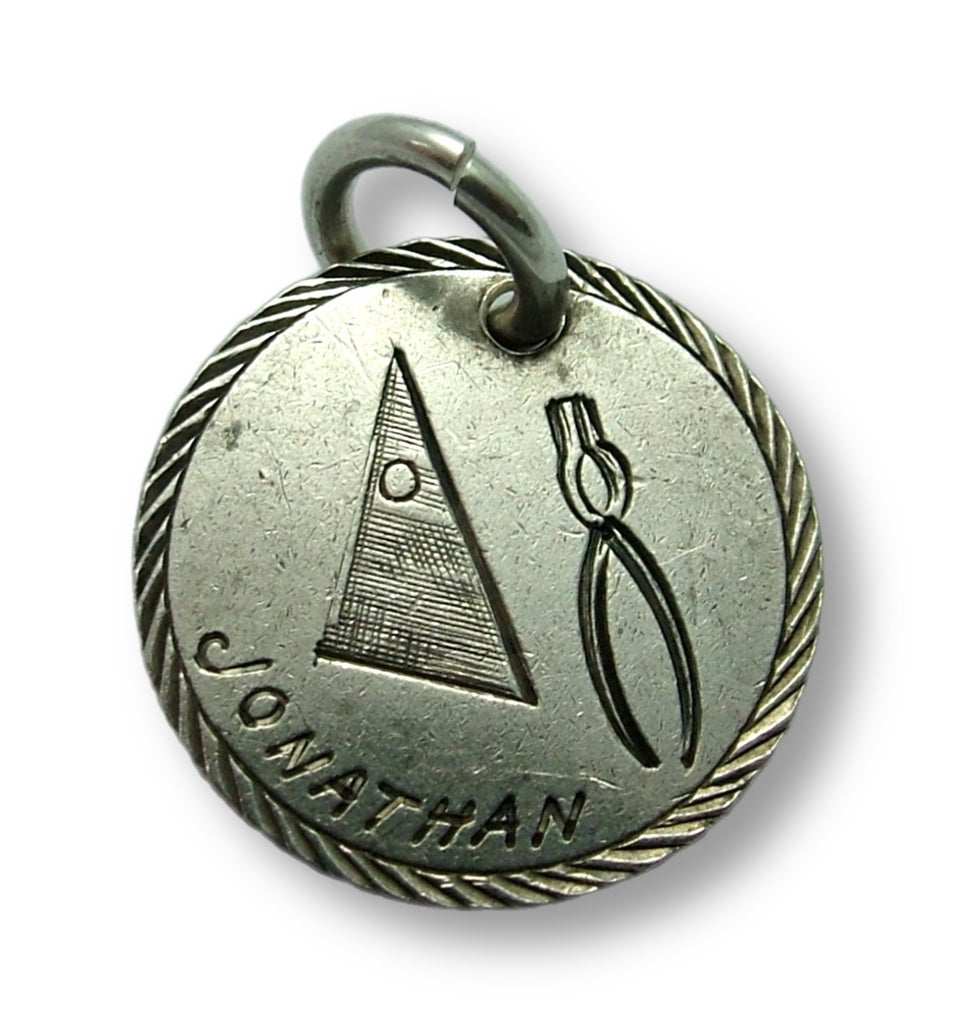The image features a round, silver medallion with a greenish tint, shown against a white background. The medallion sports a heavily engraved, circular border resembling a rope pattern, creating an illusion of motion. At the top is a visible hole containing a silver ring, designed to attach the medallion to a collar, key chain, bracelet, or tie clasp. 

In the center of the medallion, slightly tilted to the right, is a triangular engraving with an embedded small circle. The triangle is detailed with upward-tilting, hatch-mark engravings. To its right, there are engraved pliers, or tongs, with the handles extending across the lower right area of the medallion. Additionally, multiple lines radiate at angles on both the left and bottom sections of the medallion.

The name "Jonathan" is etched in a semi-circular pattern across the bottom, aligning with the medallion's curvature. The intricate details and metallic finish suggest a finely crafted piece designed for aesthetic as well as functional use.